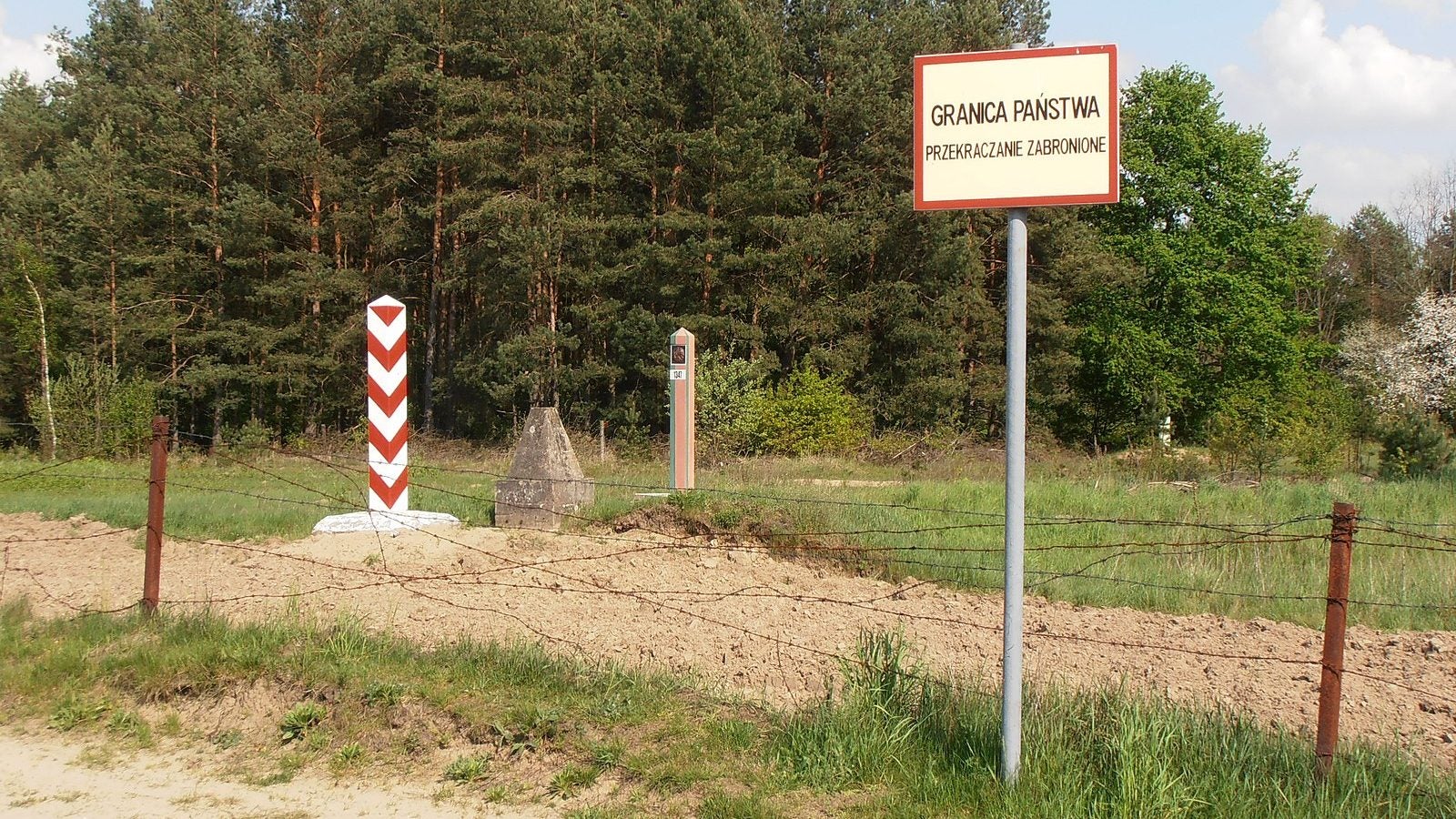The photograph captures a protected border or barrier, likely in Poland, signified by a distinctive sign in the foreground. The sign reads "Granica Państwa, Przekraczanie Zabronione" against a white background with a red border, indicating "State Border, Crossing Prohibited." The scene is set on a bright, clear day, with a light blue sky peppered with various white clouds occupying the top corners of the image.  

In the forefront, the bottom left corner reveals a sandy path that appears to be a road. Adjacent to this path is a thin strip of overgrown green grass, which is encroaching upon a barbed wire fence fixed to metal poles. This fence separates the foreground from a gravel dirt path lying just beyond it. Positioned to the left center of the image is a second post, painted in red and white, adjacent to a conical concrete slab, hinting at further demarcation. 

Behind these elements, the landscape extends into greener areas, possibly featuring large trees. Another distant post, with indistinguishable colors possibly of blue and pink hues, is also visible but too far to discern any specific details. The overall composition suggests a well-guarded and clearly marked boundary, with multiple elements reinforcing its protected status under the wide, sunlit sky.